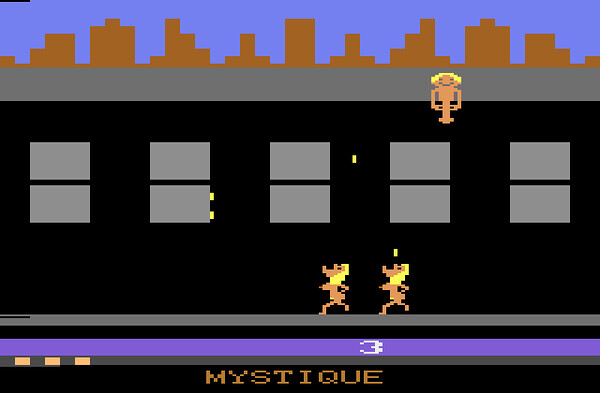This image is a screenshot from an old-school style video game, likely reminiscent of retro Atari games. Dominating the screen is a mostly black background, with an array of ten gray rectangles, resembling windows, spaced in pairs horizontally. Situated at the bottom of this display are two female avatars with blond hair, heads tilted back, and mouths open as if catching small, yellow blocks being dropped from above. Both avatars are depicted nude, featuring simple pixelated graphics. Above them, perched on top of what appears to be a large black building, is another male avatar, also nude, seemingly dropping these yellow blocks. The skyline behind this male avatar includes a silhouette of buildings against a blue backdrop, providing a sense of depth. At the bottom of the game screen, in orange font, the title "Mystique" is displayed, along with the number three, possibly indicating the level or score.